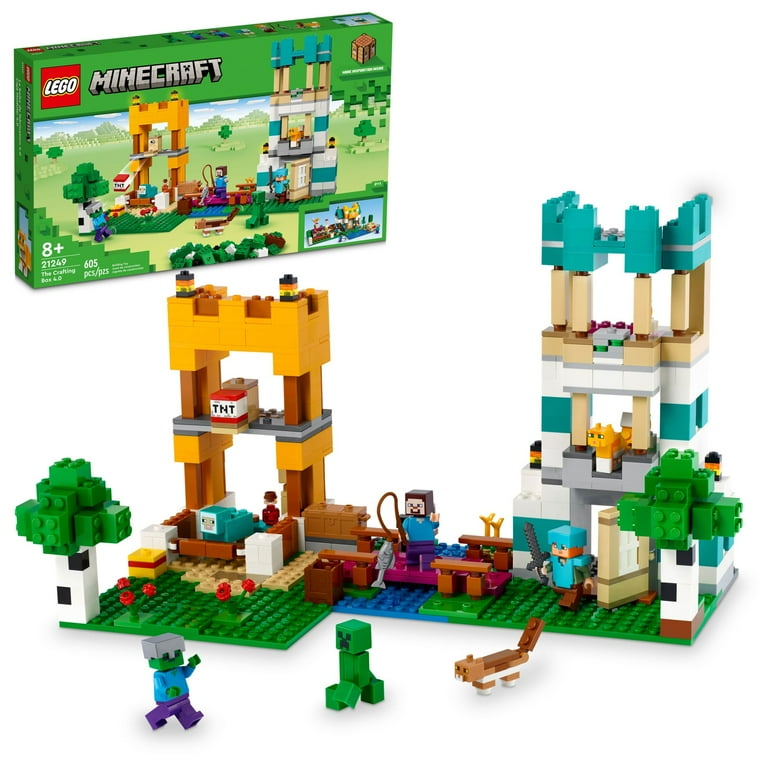This image showcases a detailed Lego Minecraft set assembled to depict a dynamic scene. In the upper left corner, the green Lego Minecraft box is prominently displayed, illustrating the same scene constructed below. Just beneath the box, the assembled Legos recreate a lively setting: two structures flank the scene, one on the left made of orange and brown bricks, and another on the right composed of aqua, yellow, and white pieces. The ground beneath is a flat white surface.

In the central area, a key feature is a man standing on a bridge, engaged in fishing. To his left, a tree and a small building are visible. Exiting the door of the structure on the right, a man wearing a light teal shirt and hat is holding a gray sword. Right below are two creatures: a green being with gray hair and a four-legged green creature. Further to the right, there is a brown and tan squirrel-like animal with white feet.

Overall, the image captures a vibrant, miniature Minecraft world meticulously assembled from Legos, with various figures and animals populating the distinctive, colorful landscape.